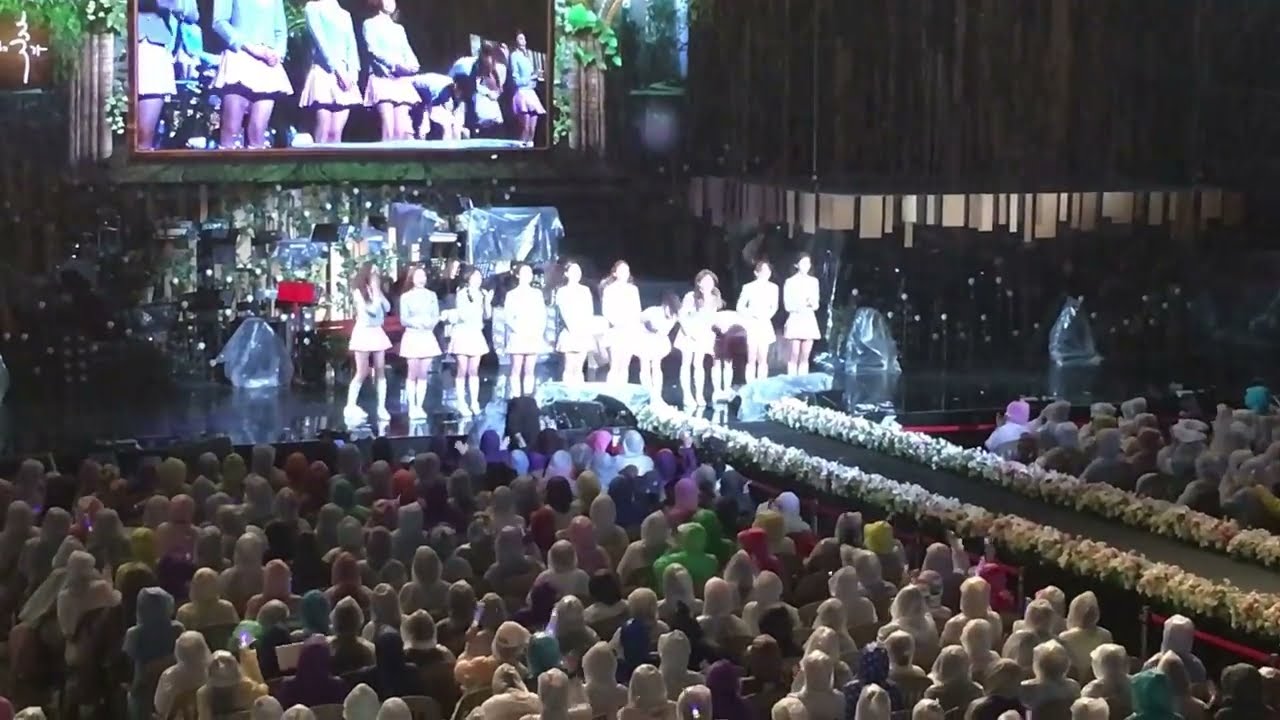The image captures a vibrant scene from a K-pop concert, featuring an all-female group of performers who seem to be expressing gratitude post-performance. The stage is set outdoors, evidenced by the audience members donning raincoats and plastic coverings on and around the stage, indicating a rainy setting. There are 10 to 11 female performers, all dressed in coordinated outfits featuring white short skirts, either white boots or tall white socks with white shoes. The stage is flanked by audiences on both sides, with a narrow runway adorned with flowers running down the center. Above the performers is a large video screen displaying a close-up view for better visibility. Bright spotlights illuminate the scene, capturing the excitement and energy of the performers, who appear happy and enthusiastic. Additional stage equipment, such as speakers, is also visible in the background, contributing to the concert atmosphere.